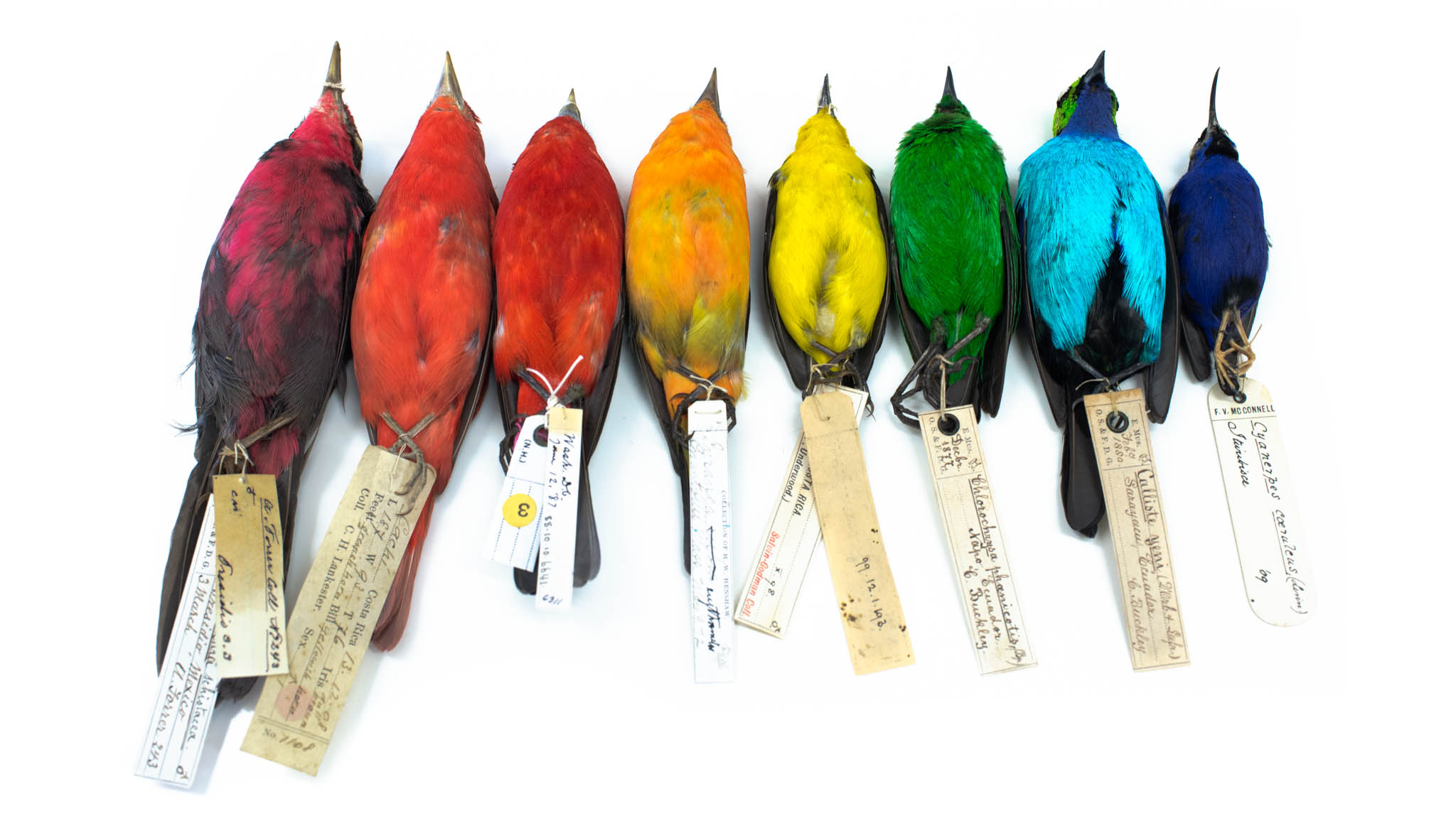This image showcases a meticulously arranged collection of taxidermied birds, each with a tag hanging from their legs, indicating their species and possibly their names, though the writing isn't clearly visible. The birds are laid on their backs against a pristine white background, with their beaks pointing upwards and tails downwards, creating a uniform presentation. The collection comprises eight birds, sorted by color to mimic the spectrum of a rainbow. From left to right, we have a large bird with deep red and black feathers and a thick, moderately long beak, followed by a reddish-orange bird with a shorter pointed beak. Next is a slightly smaller bird with deeper red feathers and a thinner, pointier beak. Proceeding to an orange bird tinged with green, having a moderately thick, pointy beak. Then there is a yellow and black bird, the smallest of the group, yet with a prominently long, pointy beak. Following it is a green and black bird with a thin, pointy beak. The second largest bird, decked in light blue and black, has a shorter but thicker beak. Finally, the sequence concludes with a dark blue bird sporting a remarkably long, pointy beak. The birds vary slightly in size, but the dark blue bird to the far right is the smallest overall. Each toe tag, dangling below the birds, adds a touch of scientific authenticity to this vivid and carefully crafted display.